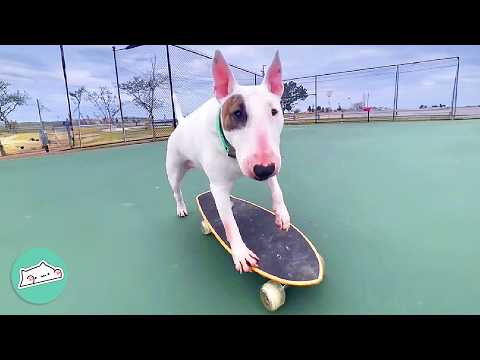A white Staffordshire Bull Terrier with pointy pink ears and a rosy snout, featuring a distinct dark patch over his left eye, is captured in this daytime photograph. The dog is positioned on a black skateboard with yellow trim and two visible wheels. His right front paw and left rear paw rest on the skateboard, while his right rear paw is on the ground and his left front paw is raised. The scene takes place in a fenced area of a sports section in a park, likely designated for activities such as tennis, judging by the green prepped surface. In the background, a chain-link fence encloses the area, and beyond it, sparse trees and a flat landscape with distant buildings are visible. The dog is staring straight at the camera, adding a sense of engagement to the image. Additionally, a logo resembling a cat or animal appears in the lower left-hand corner of the photograph. Clouds can be seen in the sky, indicating that the photo was taken during the day.